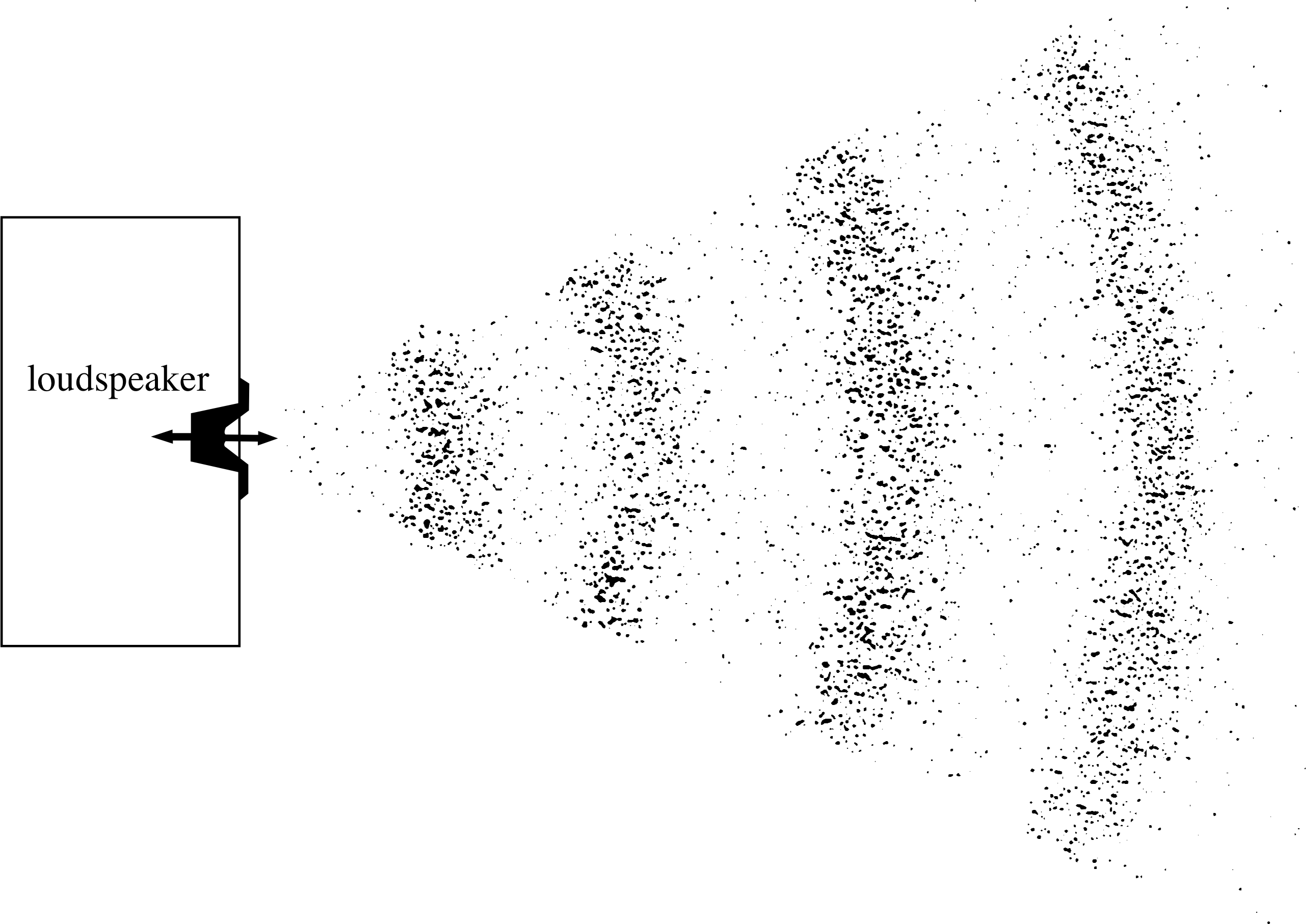In this simplistic black-and-white image, the background is predominantly white with black elements forming a detailed diagram. To the left of the image, there's a vertical rectangular box labeled "loudspeaker" in lowercase black text, slightly above the center. On the right side of this rectangle is a small, solid black shape attached to a double-ended arrow extending through this shape; one end of the arrow points towards the loudspeaker while the other extends outward. From this arrow, a series of black dots radiate outward in a cone-like pattern, resembling the shape of a piece of pie with the tip pointing towards the loudspeaker and the wider end spreading outwards. These dots alternate between closely packed and more spaced-out clusters, visually representing the transmission of sound waves from the loudspeaker, expanding until they reach the top left, top right, and bottom right corners of the image.